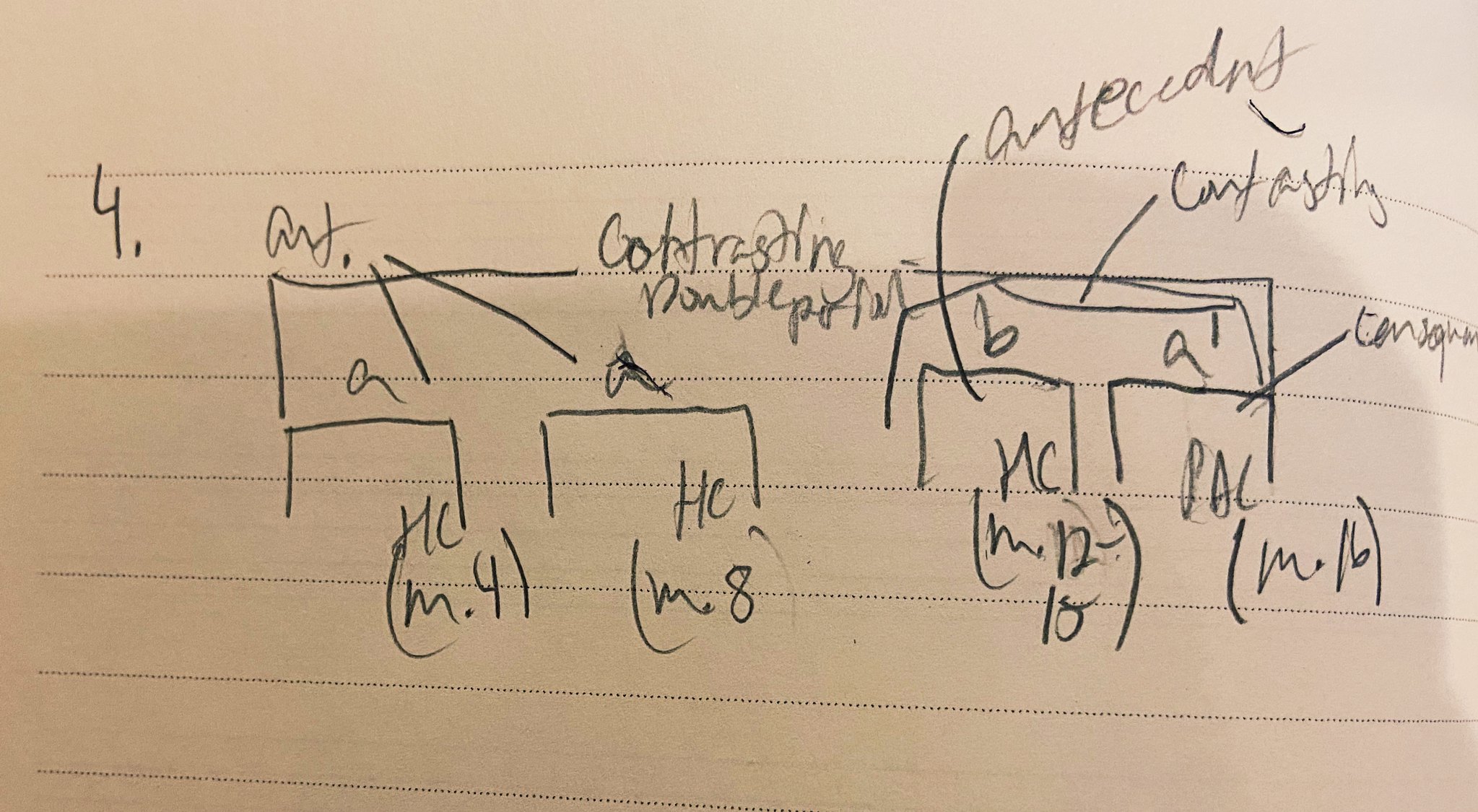Close-up of a handwritten note in a light tan notebook with small, dotted demarcation lines that create the illusion of horizontal writing lines. The note pertains to problem number 4 and is crafted in black ink. At the top, difficult-to-read writing occupies the first line. Below this, a detailed diagram featuring a vertical flow suggests a causal relationship among various components. The diagram includes multiple boxes and staple-like shapes connected in a top-to-bottom sequence.

Visually divided into left and right sections, this diagram might be illustrating different scenarios or effects. In both sections, staples are labeled either "A" or "B" on the second line. Further down, each of the four staple-like shapes in both halves is marked with "HC." Parenthetical notations, such as M.4, M.8, M.12, M.18, and M.16, are written from left to right beneath these staples, indicating a possible sequence or categorization. The structured layout and annotations suggest a methodical approach to solving a complex problem.